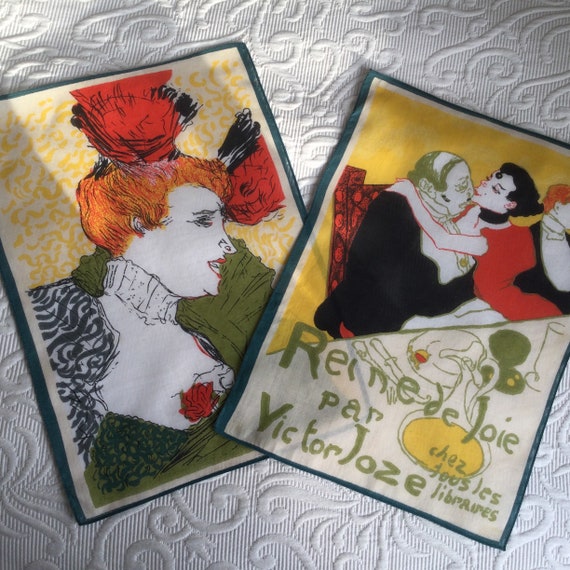This photograph features a pair of rectangular napkins or pieces of fabric, each adorned with intricate designs and laid on a white, filigree tablecloth or bedspread. Both napkins are about the size of a card and are bordered in black. They each display scenes with people dressed in old-fashioned clothing. The piece on the left shows a woman with vibrant orange hair, wearing green attire and appearing to have a headache. Meanwhile, the piece on the right depicts a man in a black jacket kissing a woman dressed in red. The figures are reminiscent of a bygone era, complete with elaborate hairstyles and accessories like chokers for the women and formal black suits for the men. The napkins also feature text in a foreign language, reading "Rene de Joy par Victor de Jose de Jules Lebrun."